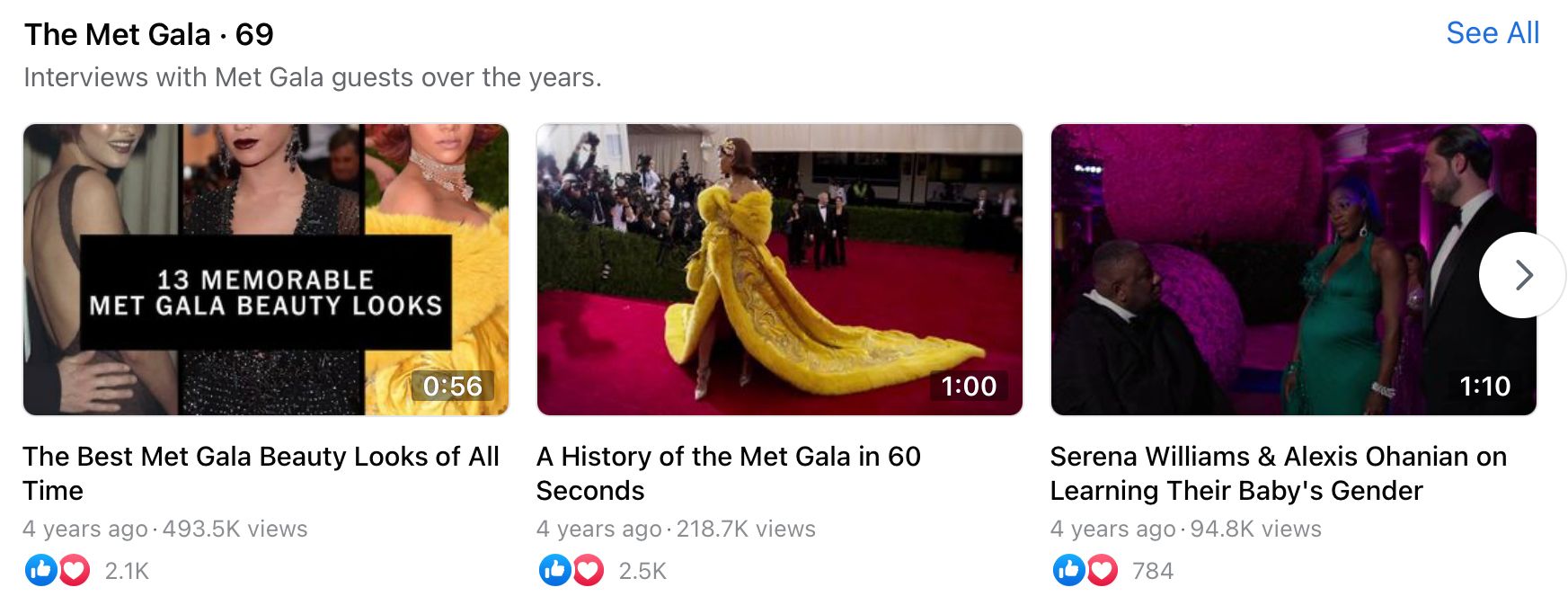**Screenshot of a Met Gala Web Page**: 

The screenshot captures the homepage of a website dedicated to Met Gala photographs. At the top center of the screen, three rectangular photos are aligned horizontally, showcasing iconic moments from the event.

- **Left Photo**: A close-up of three women, shown from mid-face to their hips. The woman on the left is dressed in a black, low-cut back dress. The center woman is also in a black dress facing forward, while the woman on the right wears a yellow dress, facing to the right. A banner across this photo reads, "13 memorable Met Gala beauty looks." Below it is the caption, "The best Met Gala beauty looks of all time. Four years ago, 493.5k views."
  
- **Center Photo**: Features a single woman standing on the red carpet in a long yellow evening gown with an extended train trailing to the right. She is facing left. The caption below reads, "A history of the Met Gala in 60 seconds from four years ago, 218.7k views."

- **Right Photo**: Depicts three individuals. A man on the left, dressed in a black suit with a white shirt, is facing left. The woman at the center, who appears pregnant, wears a green evening gown. She has dark skin and her hair is styled in an updo. To the far right, another man in a black suit with dark skin and very short hair stands. The caption beneath states, "Serena Williams and Alexis Ohanian on learning their baby's gender from four years ago, 94.8k views."

Additionally, a text on the left side of the page says, "The Met Gala, 69 interviews with Met Gala guests over the years," with an option in the upper right corner that reads, "See all."